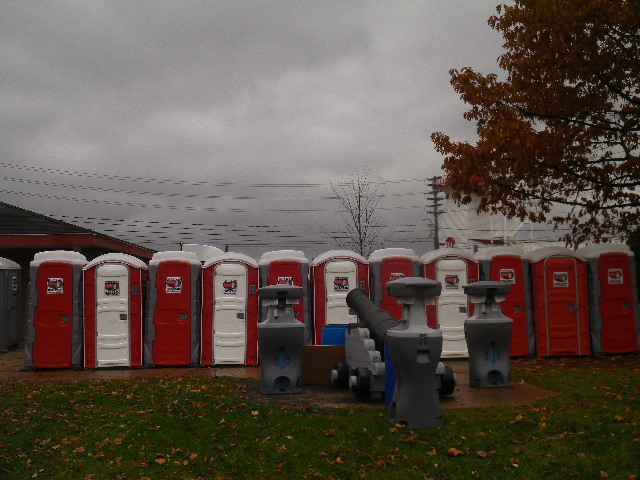The photograph, taken outdoors on a stormy, gray day, features a grassy foreground scattered with brown leaves. At the front center, a detailed trash can with a gray base, slim neck, and flat top stands on a concrete surface, flanked by similar trash cans to the left and right. Behind these trash cans, an iron structure resembling a cannon on four black wheels points upward, positioned centrally among the port-a-potties. These port-a-potties, numbering ten, are arranged in varying colors of gray, red, and white, alternating in sequence except for the last three, which are all gray and red. Midway up the image, intersecting power lines extend across the scene from a green-roofed building on the left. A barren tree without leaves punctuates the skyline, while an autumn-colored tree with reddish-brown leaves stands prominent on the right.